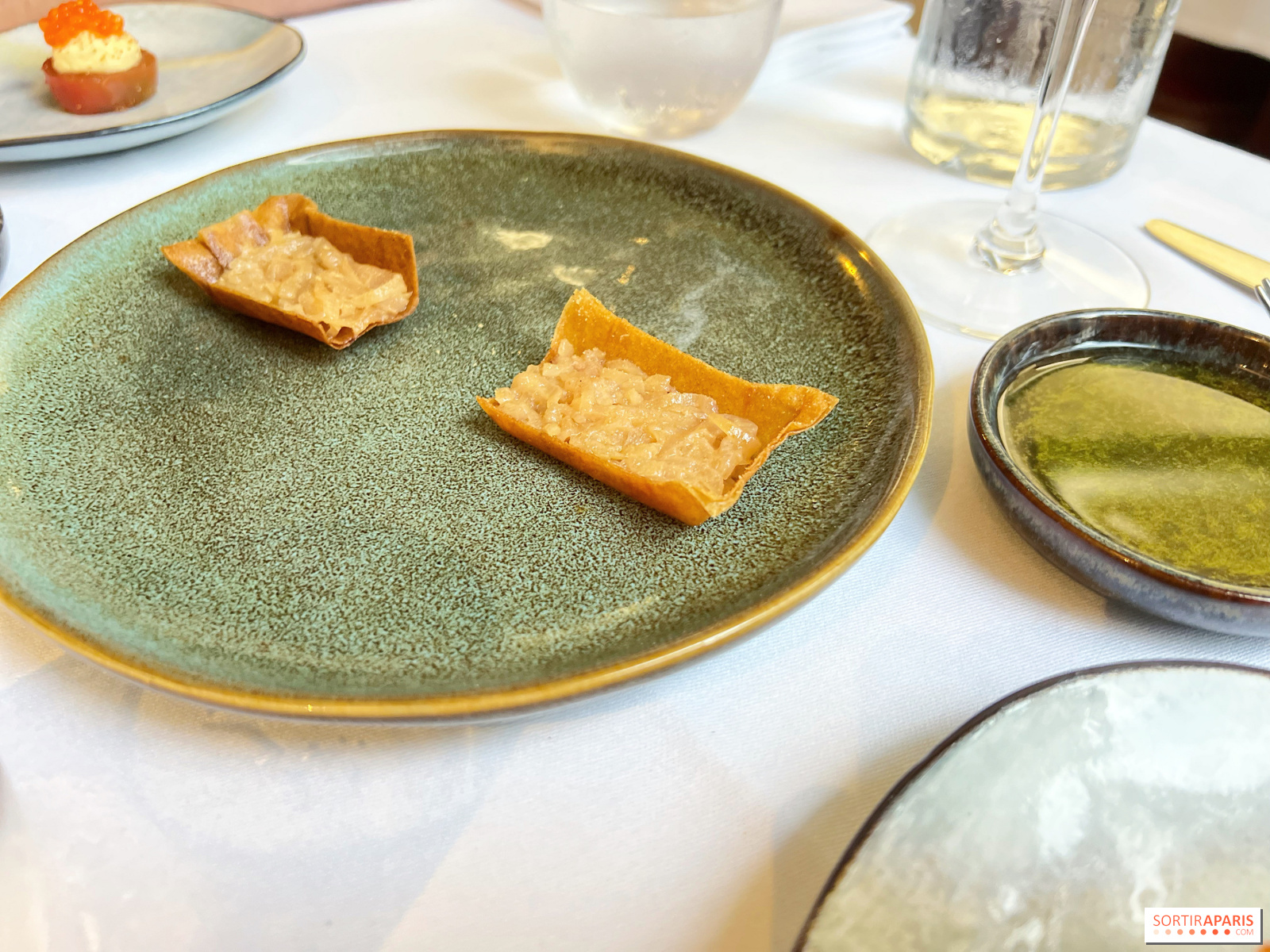The image depicts a well-lit dining table with a green plate bordered in yellow at the center. This plate features what appear to be two crackers or possibly a single cracker broken in half. Nearby, on the same table, is a nearly empty pitcher with a small amount of yellow liquid at the bottom. Below the green plate, there's a shallow blue bowl filled with something green that covers the bowl's base. In the lower right corner, an empty white plate is visible. To the upper left, a white plate holds a couple of unidentified stuffed items, resembling stuffed apricots. There are also reflections and shadows cast on the white dining table. Additionally, a watermark reading "Sautiuraparis.com" appears at the bottom right corner of the image, adding a touch of stylistic branding. Various table elements including a knife, wine glass stem, and water pitcher are also included, suggesting a recently finished meal.